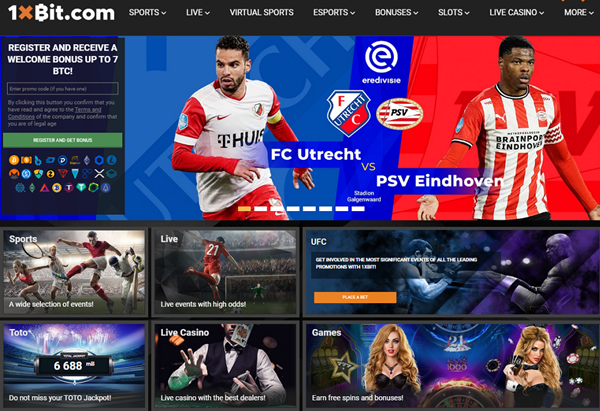*Detailed Caption for the Image:*

The image appears to be an advertisement or homepage for a betting website, featuring a dark background. In the top left corner, there's a logo consisting of a white figure followed by an orange 'X' and the text 'bit.com' in white. To the right of the logo, several menu options are listed in white text: Sports, Live, Virtual Sports, Esports, Bonuses, Slots, Live Casino, and more. A prominent promotional message reads, "Register and receive a welcome bonus up to 7 BTC."

On the left-hand side, a green box with white text (not legible) is visible, accompanied by numerous small icons that appear to represent different cryptocurrencies, possibly various types of Bitcoin. 

The central part of the image features a picture of two male soccer players in jerseys. The player on the left wears a predominantly white jersey with red sleeves, while the player on the right sports a red and white striped jersey. Text below the players identifies a match between FC Utrecht and PSV Eindhoven.

Below this, several rectangles highlight different sections and promotions available on the website:
- A section labeled "Sports" shows an image of a soccer match with the description, "Wide selection of events."
- Another section titled "Live" features a soccer match image and mentions "Live events with high odds."
- The "UFC" section displays two fighters standing beside each other.
- "Toto 6688" promotes a jackpot with the phrase, "Do not miss your Toto jackpot."
- The "Live Casino" section shows a head-and-shoulders image of a man in a waistcoat and bow tie throwing cards in the air.
- A section titled "Games" displays two blonde women in black corsets, one with a bow tie and the other with a black necklace, alongside a roulette wheel. The text here mentions "Earn free spins and bonuses."

Overall, the image illustrates various betting options and promotions, indicating that it is indeed a betting website.